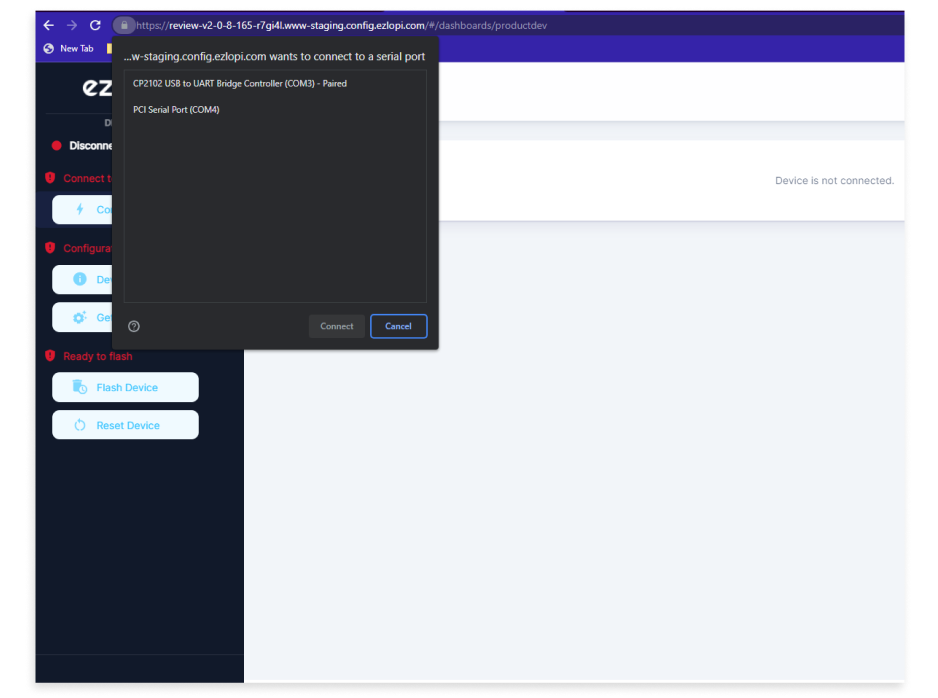This image is a screenshot of a web browser displaying a web page. The URL is a long, secure HTTPS address, indicated by a padlock icon in the address bar. The padlock icon has been clicked, revealing a pop-up box prompting the user to connect to a serial port, with two serial port options listed. This black pop-up box obscures a portion of the website content.

On the left side of the webpage, there is a navigation menu featuring options related to "Connecting," "Configuring," and "Ready to Flash," which appear to pertain to flashing devices. The main section of the webpage has a grey background. A white text box in the center of this section bears the message "Device is not connected" in grey text. Apart from this navigational menu and the text box, the rest of the webpage is blank.